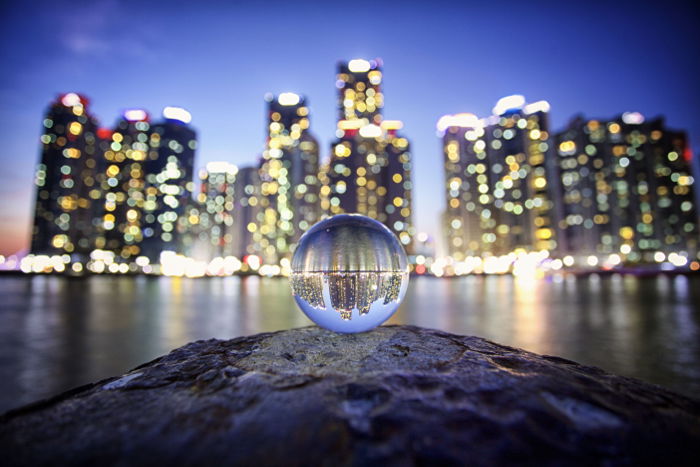This photograph captures an artistic and abstract scene of a nighttime city skyline reflected in a clear, spherical glass orb. The orb, resembling a large raindrop, sits atop a rugged rock formation overlooking a tranquil lake. Within the reflective surface of the orb, the cityscape appears inverted and slightly distorted, showcasing tall, dark-skinned skyscrapers with illuminated windows that emit a yellow lens flare effect. Bright white dots near the base of the buildings suggest bustling city streets. The lake separating the rock from the city is serene and almost mirror-like. The sky transitions from light blue to darker hues, interspersed with shades of pink, indicative of a sunset or twilight setting. The edges of the image are vignetted, adding a subtle black fade towards the corners, enhancing the overall dreamy and abstract quality of the photograph.